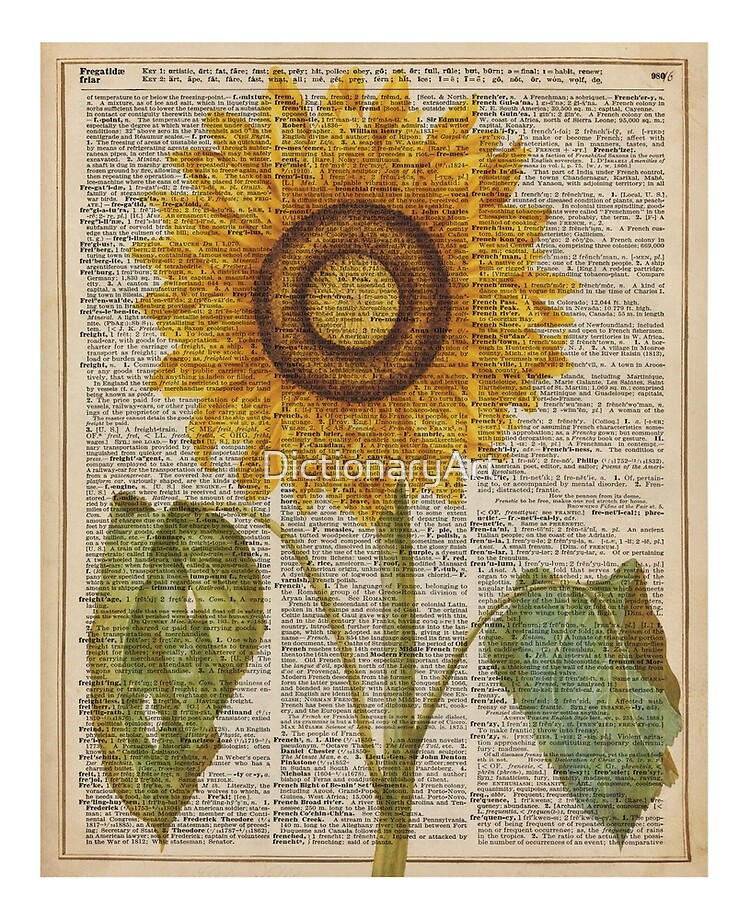The image showcases a vibrant sunflower with bright yellow petals encircling a dark brown center, resembling a large, detailed donut. The sunflower stands prominently against the textured, beige page of an old dictionary, featuring three long vertical columns of black text, each beginning with bolded words starting with the letter 'F'. The detailed illustration of the sunflower includes a green stem and two large leaves at the bottom left and right, with the left leaf appearing more tattered with holes. Superimposed across the image, in faded white letters, is the phrase "Dictionary Art," adding a modern touch to the vintage backdrop. The entire composition blends botanical beauty with antique textual charm, making for a striking piece of art.